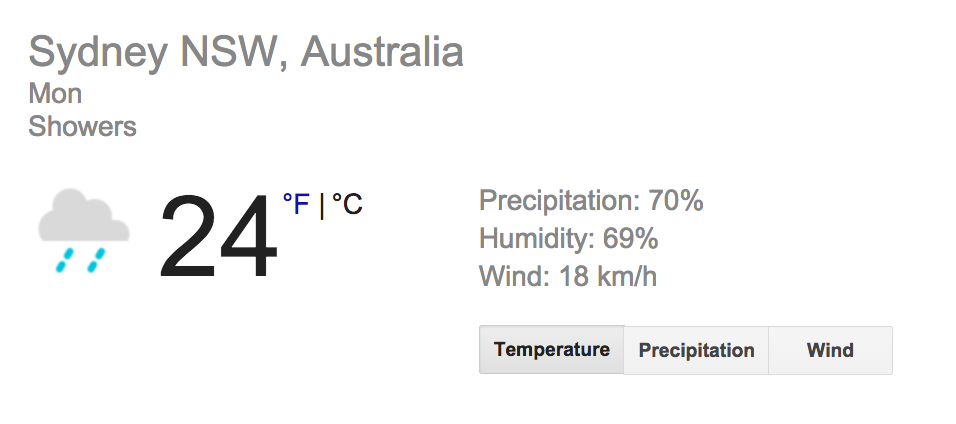The image displays a digital weather report for Sydney, NSW, Australia. The background is white, and at the top, in grayprint, it reads "Sydney, NSW, Australia." The next line indicates "Mon" for Monday, followed by the word "showers." On the left side of the image, there is a gray cloud icon with blue lines representing rain. Next to the cloud icon, in black print, the temperature is shown as "24°" and includes both Fahrenheit and Celsius options, though Sydney typically uses Celsius.

Toward the right side, the report details the weather conditions with "Precipitation: 70%," "Humidity: 69%," and "Wind: 18 km/h." At the bottom of the image are clickable rectangular buttons labeled "Temperature," "Precipitation," and "Wind."